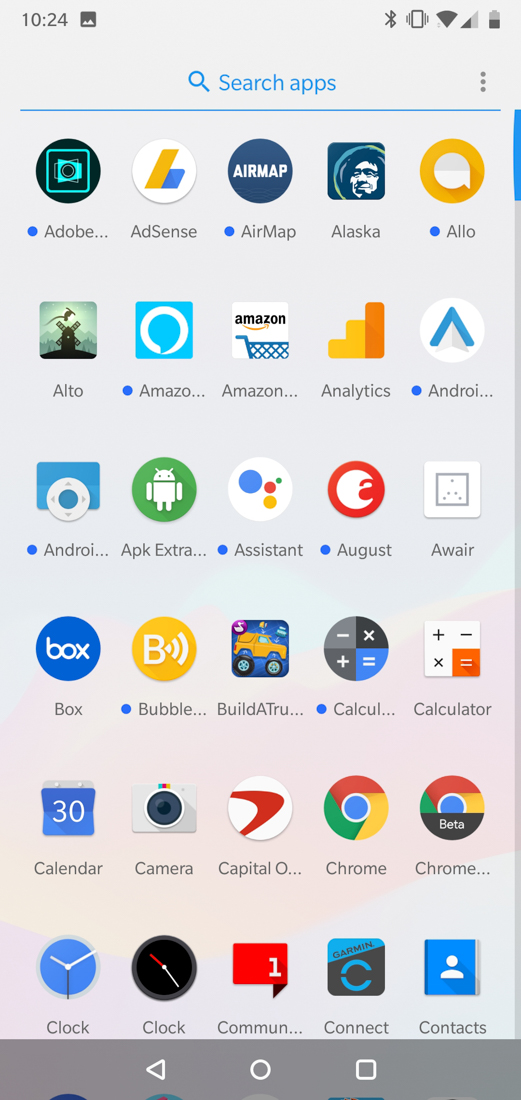This image showcases a smartphone screen displaying a 5x5 grid of app icons, arranged in alphabetical order. The visible apps include Adobe, AdSense, AirMap, Alaska, Allo, Alto, Amazon Alexa, Amazon Shopping, Analytics, Android System, APK Extractor, Assistant, August, Aware, Box, Bubble Level, Build-A-Truck, Calculator, Calendar, Camera, Capital One, Chrome, and Clock. A search bar is positioned at the top of the screen against a light gradient background. The screen's status bar reads 10:24, indicating the time, and displays icons for full Wi-Fi signal, half cellular service, active Bluetooth, vibrate mode, and a battery that is approximately halfway charged. Below the app grid, the standard Android navigation buttons for back, home, and recent apps are visible. It is evident that there are more apps beyond the initial viewable grid, as suggested by the scrolling indicator.